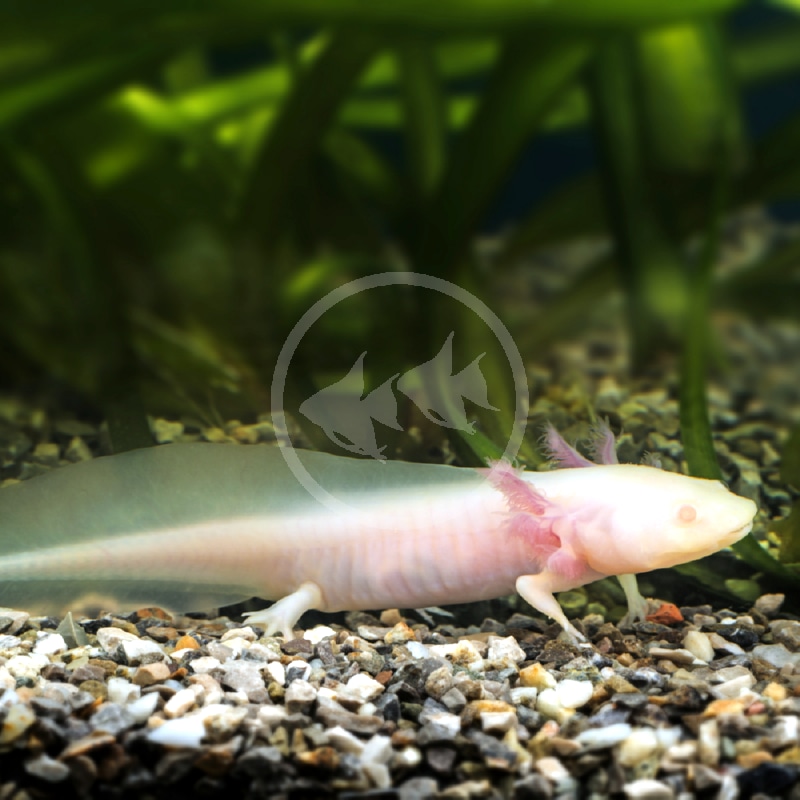The photograph showcases a young axolotl, a distinctive amphibian native to Mexico, situated in an aquatic environment that resembles an aquarium. The creature, slightly pink with nearly translucent skin, sits on a gravelly bed surrounded by small vegetation and various plants in the background. Characteristic of axolotls, it has a long, finned tail and feathery, purple gills protruding from either side of its head, reminiscent of delicate tentacles. The setting, likely a fish tank or similar container, also features a watermark depicting two fishes swimming in a circular pattern on the lower part of the image.